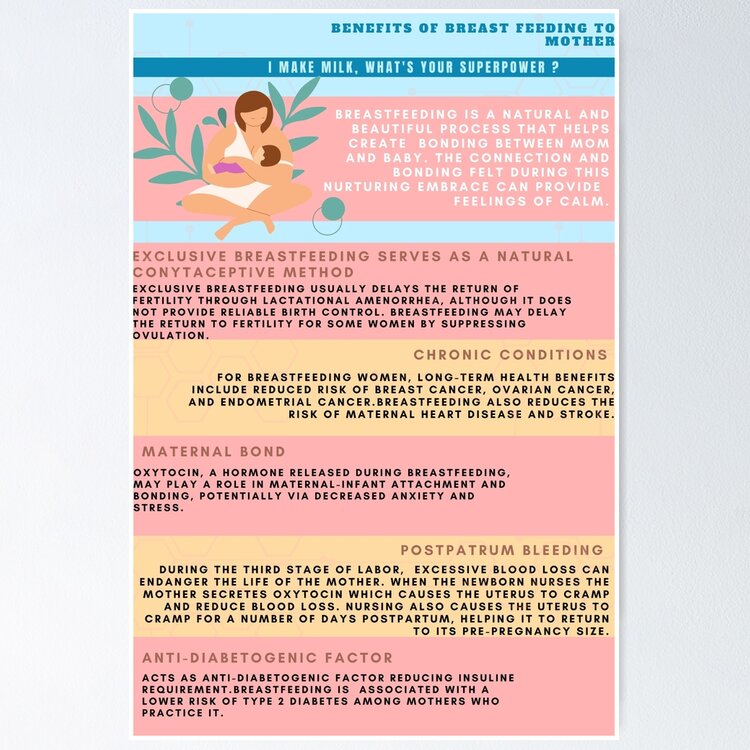The flyer, bordered in white, is designed with alternating strips of light blue, dark blue, pink, and orange-yellow, each section containing informative text. At the top, within a light blue section, the dark blue text reads, "Benefits of Breastfeeding to Mother." Directly below that, a thin dark blue banner states, "I make milk, what's your superpower?"

The main visual feature of the flyer is a cartoon-like illustration of a mother breastfeeding her child. She has short brown hair, wears a white dress with one shoulder pulled down, and sits cross-legged, surrounded by plants. The infant, also with short brown hair, is dressed in pink.

Accompanying the illustration is the text: "Breastfeeding is a natural and beautiful process that helps create bonding between mom and baby. The connection and bonding felt during this nurturing embrace can provide feelings of calm."

Further down, the flyer is divided into five sections, each emphasizing different benefits of breastfeeding. These sections are titled:

1. "Exclusive Breastfeeding Serves as a Natural Contraceptive Method."
2. "Chronic Conditions: Long-term health benefits include reduced risk of breast and ovarian cancer."
3. "Maternal Bond."
4. "Postpartum Bleeding: Nursing helps the uterus return to pre-pregnancy size and reduces excessive postpartum bleeding."
5. "Anti-Diabetogenic Factor: Reduces insulin requirements, acting as an anti-diabetic agent."

Despite a few minor typographical errors, the flyer is colorful and effectively highlights the multifaceted benefits of breastfeeding for mothers.